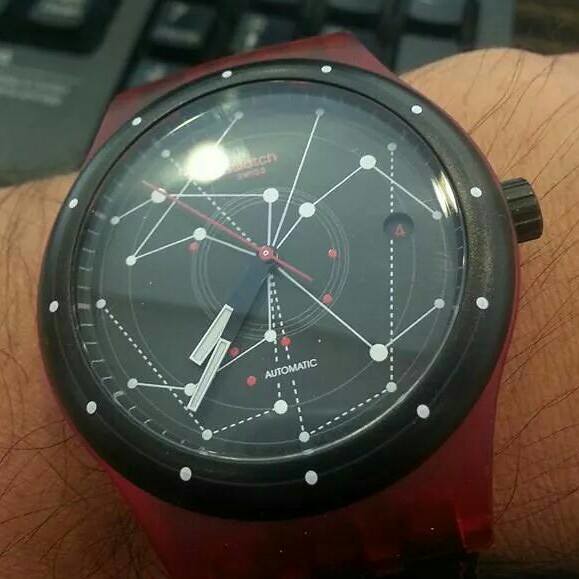This is a photograph of a distinctive watch on a man's hairy wrist, angled up towards the right. The watch is characterized by its round face, which fills almost the entire frame, and features a dark green outer ring and a lighter green center. Notably, the watch lacks standard numbers, featuring instead 12 dots and various dashes. In the middle, partially obscured by a glare, are constellation symbols and the word "automatic." The watch has two black hands with silver tips, a red second hand, and appears to be a Swatch model, indicated by the word "Swiss" under the Swatch emblem. The maroon band is made of plastic, complemented by a winding button on the right side of the watch face. The background includes indistinct elements in black and blue-green hues, with a keyboard faintly visible.